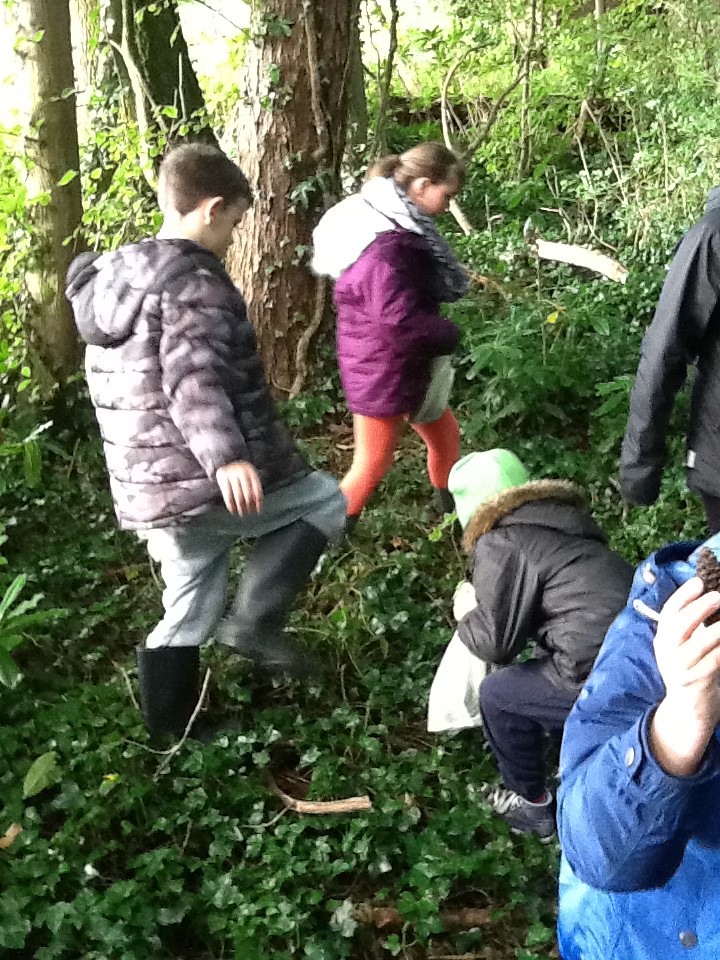In this picture, a group of individuals, potentially a family, is seen exploring a sunlit forest. They appear to be engaged in a search for something, possibly collecting items such as rocks, sticks, mushrooms, or litter. The scene captures a sense of adventure and environmental awareness. Among the group, a child in a black coat, a lady in a pink coat, and another person in a blue coat stand out. Additionally, there are three visible children, including one with a green hat and coat, who is seen reaching down into the forest, and a male child actively taking a step while looking away from the camera. Partial glimpses of other individuals, likely adults, are also visible. The group is dressed in warm but not overly heavy coats, suggesting a cool but not freezing atmosphere, underscored by the bright sunshine illuminating the background and reflecting off the trees and green vegetation. The scene conveys a serene, timeless quality and showcases an idyllic natural setting.